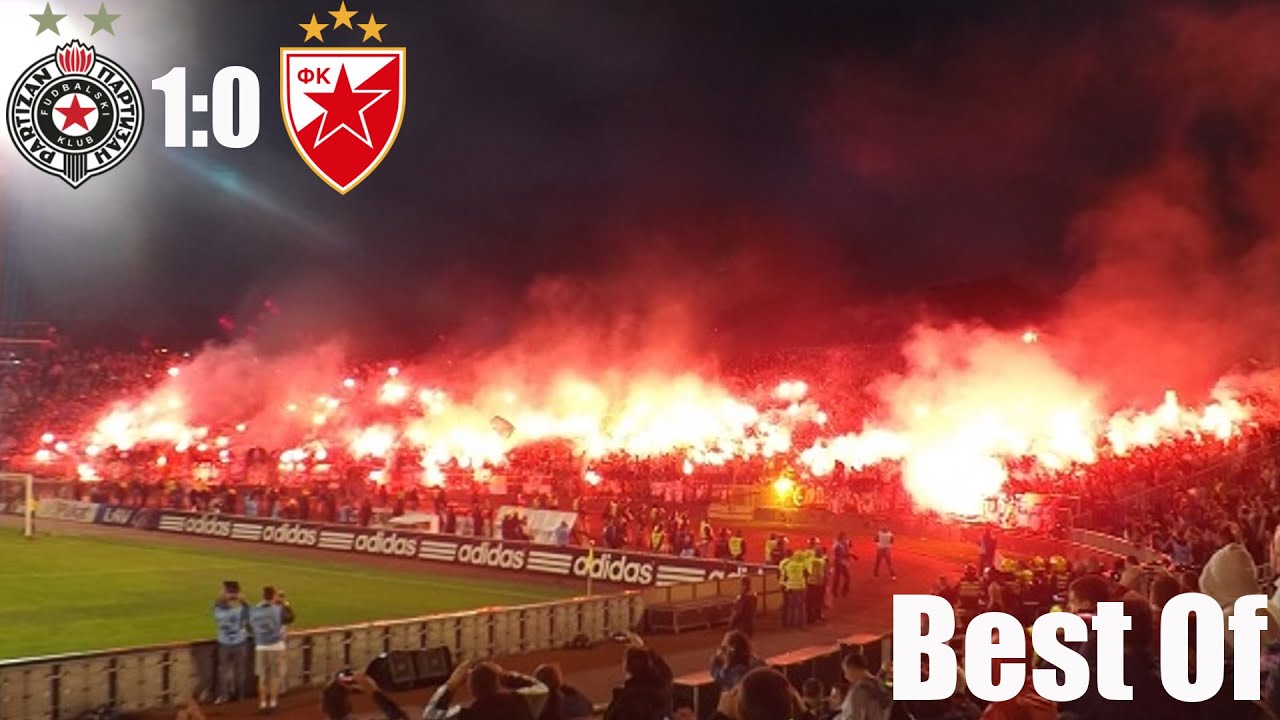The image captures a dramatic night scene within an outdoor soccer stadium, possibly during or after a match. The dark sky is illuminated by intense flames and thick smoke rising from the crowded stands, suggesting a pyrotechnic event gone wrong. The fire seems to engulf sections of the stands, creating a chaotic and alarming atmosphere. Surrounding the field, which features green turf and a white soccer goal on the left, there are visible Adidas logos on the border. A track encircles the field where numerous onlookers and security personnel are gathered, attentively watching the blaze. In the upper left corner of the image, two logos are displayed: one circular emblem with a red star and some foreign text, and a shield with a red star and three gold stars above it, indicating the teams or clubs involved, with a score of 1:0. The top left also features two gray stars. On the bottom right, in white font, the words "Best Of" are prominently displayed, adding a final touch to the intense and chaotic scene.